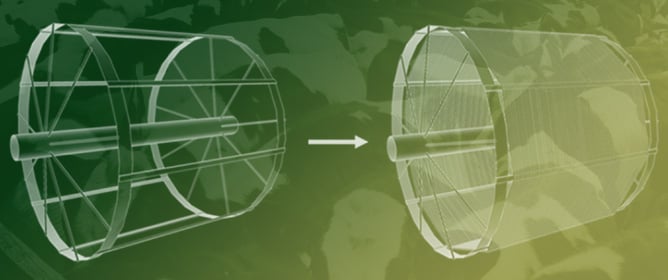The image is a detailed illustration, hazily shaded in green, depicting two cylindrical objects side by side, seemingly designed to fit into each other. The left object appears as a structural framework, resembling a wheel or fan with a central stem and radial spokes extending outward, encased in a cylindrical shape. This skeletal structure is contrasted with the right object, which shows the framework more solidified, indicating joints where sections connect. An arrow points from the left to the right, suggesting the manner in which these two objects interconnect. An additional green arrow further implies the direction of their assembly. The illustration's purpose seems to convey the process of joining these devices, possibly representing varied interpretations from mechanical fans to lampshades or even larger mechanical components such as axles or turbines, although the scale remains unspecified.